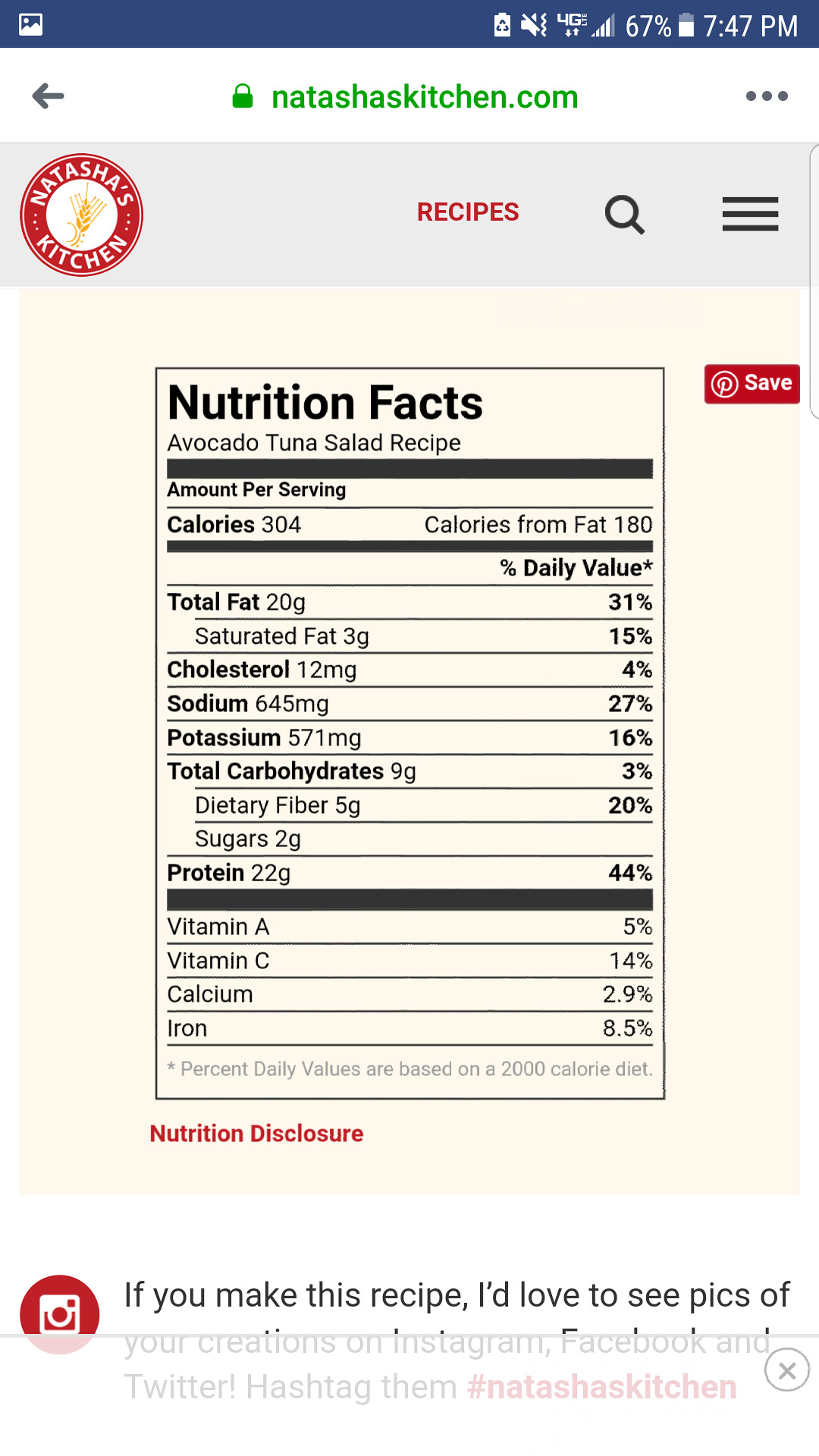A detailed screenshot from a smartphone displays a webpage from Natasha's Kitchen. At the very top of the screen, a blue status bar reveals that it is 7:47 PM and the battery is at 67%. Below the status bar, the URL natashaskitchen.com is prominently displayed, followed by a light blue navigation bar with the word "Recipes" highlighted in red. On the left side of this navigation bar is the website’s logo, consisting of a red ring inscribed with "Natasha's Kitchen," encircling a central element that appears gold but is indistinct due to the small size of the image. Dominating the majority of the screen is an image of a nutrition facts label for an Avocado Tuna Salad Recipe. Per serving, the salad contains 304 calories, 20 grams of fat, 12 milligrams of cholesterol, 645 milligrams of sodium, 9 grams of carbohydrates, 5 grams of fiber, 2 grams of sugar, and 22 grams of protein. At the bottom of the image, part of a text message is visible, inviting viewers to share pictures if they make the recipe, although part of this message is cut off and not fully legible.